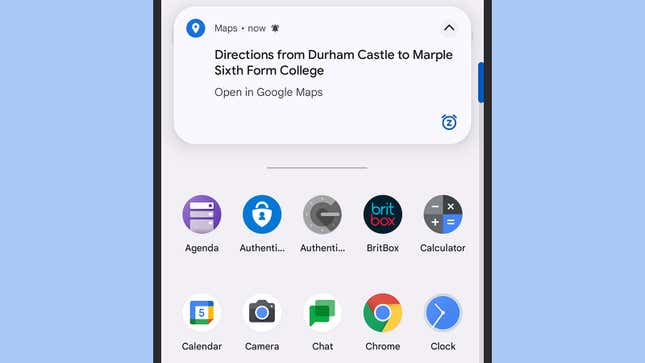The image is segmented into several distinct areas with detailed elements. 

On the left side, a light blue background occupies the first quarter of the image, bordered by a quarter-inch black line. The middle half features a light grayish background. Similarly, the rightmost quarter mirrors the left with the same light blue background and black border. 

In the central area of the image, a large white rectangle resembles a pop-up tab. In the top-left corner of this white rectangle, there is a blue circle containing a white location icon. To the right of this icon, small black text reads "Maps," followed by a dot and then the word "Now." On the right side of this bar, there is a small bell icon, and to its right, a greater-than sign pointing upwards.

Beneath the "Maps" text, bold black lettering states, "Directions from Durham Castle to Marple," followed by "6th Form College" in slightly less bold text. Below this, in smaller, less prominent text, it reads, "Opening Google Maps." In the bottom right corner of this white rectangle, there is a small blue circle with a 'Z' inside it, which resembles another bell icon.

Below this central section, a thin gray bar runs horizontally. In the middle of the image, just below this gray bar, are two rows of icons with accompanying text. The first row contains five icons and labels: "Agenda," "Authentication," another "Authentication," "Brick Box," and "Calculator." Each icon is situated above its respective label. The second row, directly below the first, includes icons for "Calendar," "Camera," "Chat," "Chrome," and "Clock," each also having its corresponding icon above it.